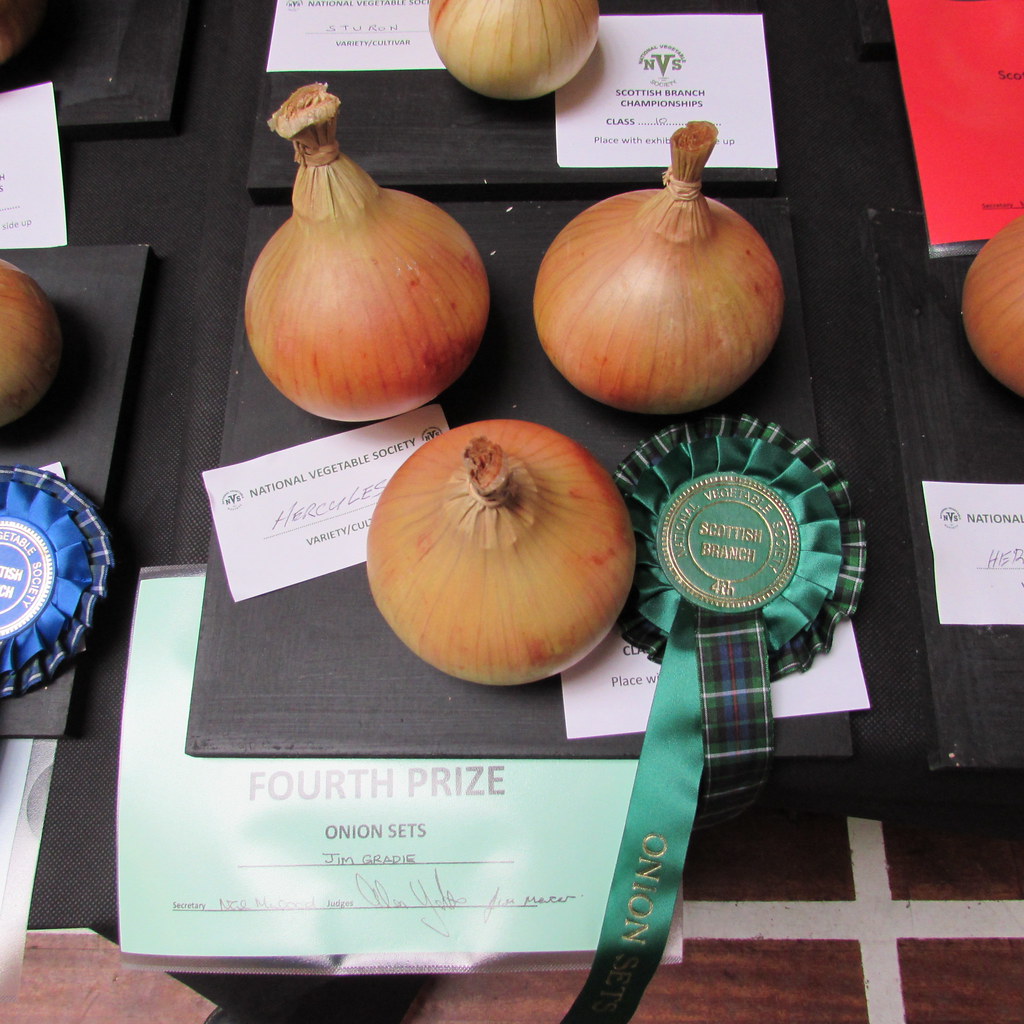The image depicts six yellow onions displayed on a black platform, partially overlapping. Three onions are fully visible while the other three are half hidden. Prominently featured alongside the onions is a green ribbon that reads "Scottish Branch" in gold lettering, with "Fourth Prize" underneath, indicating they won fourth place in an onion sets competition. The label in the middle, from the National Vegetable Society, specifies the Hercules variety of the onions. Jim Grady is the name of the participant who entered these onions into the competition. The scene suggests a setup at a vegetable show, with various tags and ribbons indicating different awards.